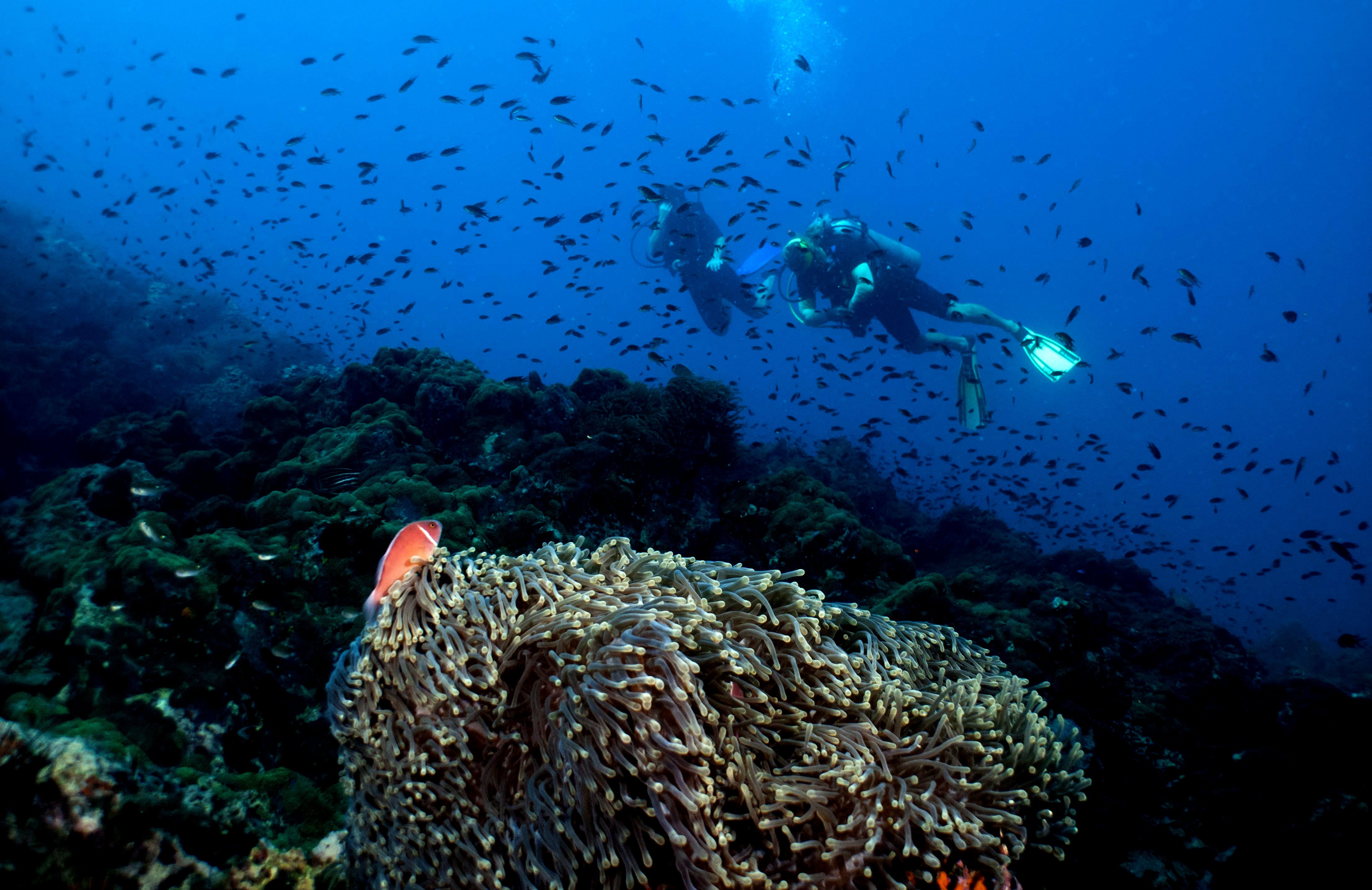In this underwater photograph, two scuba divers are seen swimming close to each other, approximately four feet apart, in the dark blue depths of the ocean. Each diver is equipped with an oxygen tank, masks, and flippers; the flippers of the diver on the left appear green, though the dark water makes the exact hue difficult to discern, while the diver on the right wears lighter-colored flippers. Both divers are dressed in very dark wetsuits, with one diver donning a short wetsuit that stops above the knees. Fish surround the scene, creating a dense, dark silhouette around the divers, except for the very top right of the image, which is almost clear. Bubbles can be seen rising from the divers in the center top of the image, adding to the dynamic underwater atmosphere. The divers are positioned above a coral reef, where a notable large orange fish with a distinctive white stripe near its head stands out, seemingly observing the divers as it looks up toward them.